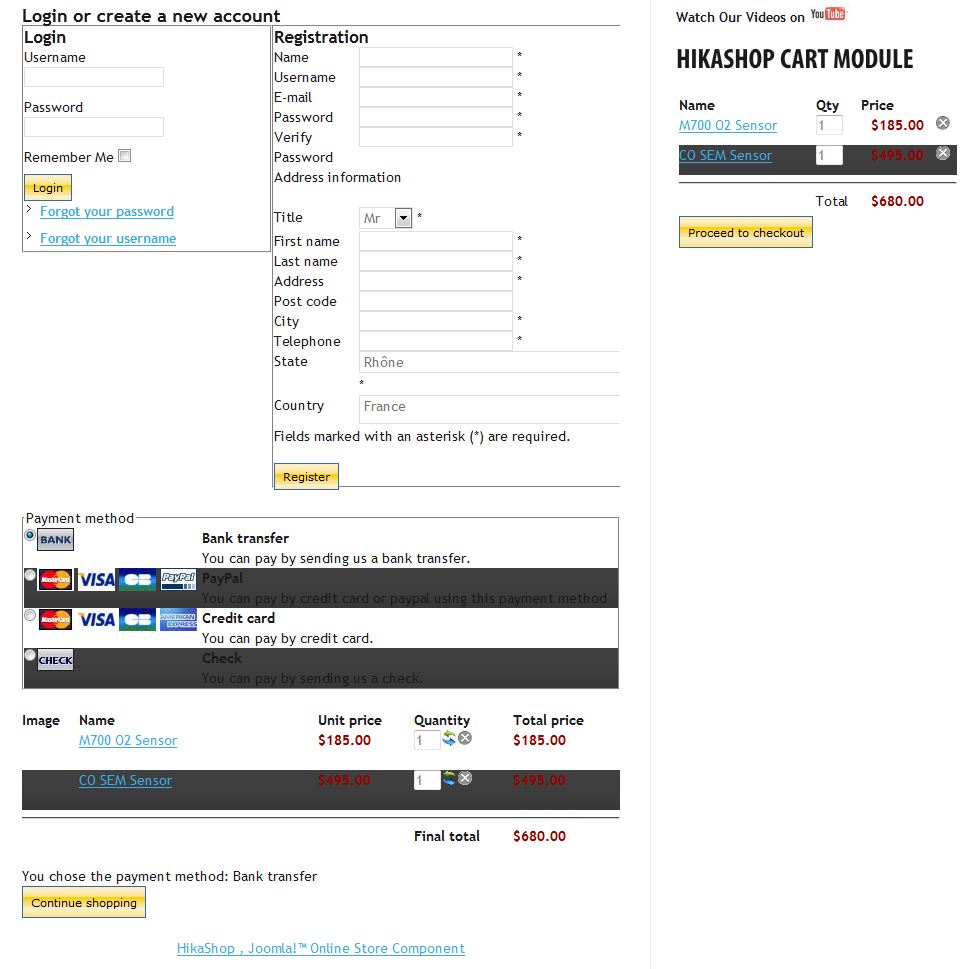This image showcases a detailed screenshot of a shopping cart module from a website. In the top right corner, the link “Watch our videos on YouTube” is visible, indicating additional support or promotional content available on YouTube. The shopping cart, named "Heika Shop Cart Module," contains two items: an M7002 sensor priced at $185 and a COSEM sensor valued at $495, making the total cost $680.

The cart interface features a prominent gold "Proceed to Checkout" button. On the left side, there are sections for "Login" or "Create New Account." The login area includes fields for the username and password, with options to remember the user and buttons for logging in or retrieving a forgotten username or password. Adjacent to the login section is a registration box asking for the typical details required to create a new account.

At the bottom of the image, the payment method section presents various options: bank transfer, PayPal, credit card, and check. The user has currently selected "Bank Transfer," with details noting, "You can pay by sending us a bank transfer." The area reconfirms the total amount payable along with the item list, quantities, and prices. Additionally, there is an option to continue shopping.

The overall interface suggests a well-organized e-commerce platform with various functionalities for a seamless shopping experience.